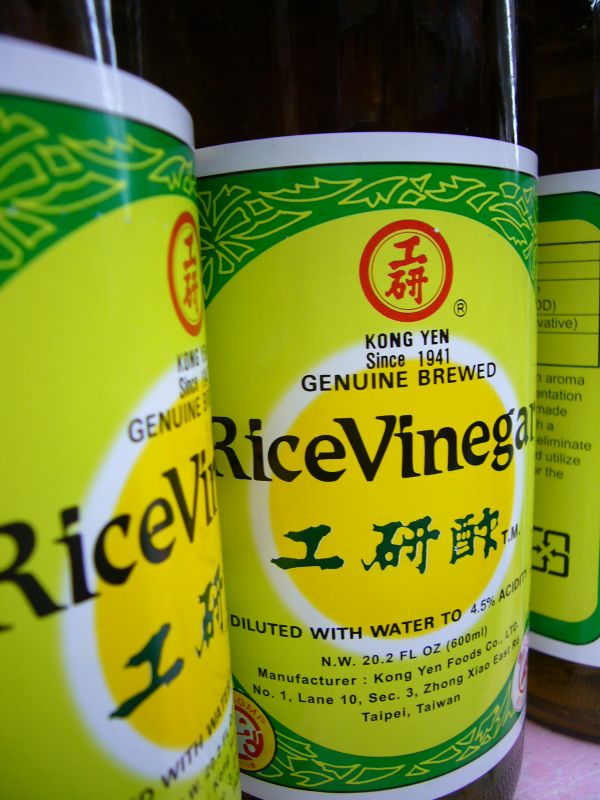The close-up photo features three bottles of Kong Yen genuine brewed rice vinegar, prominently displaying the front label of the center bottle. The label, predominantly green with decorative elements, includes a lime green circle with a yellow center and black text stating "Rice Vinegar" and "diluted with water" with 4.5% acidity. Above the text, there's a red Taiwanese character, and the bottom of the label notes its origin: Taipei, Taiwan. The white, yellow, and various green shades enhance the packaging. The white-capped bottles are aligned neatly, showcasing the brand's heritage, "Kong Yen, since 1941," from the genuine brewed label to the manufacturer, Kong Yen Foods Co., on the shelves of a store.